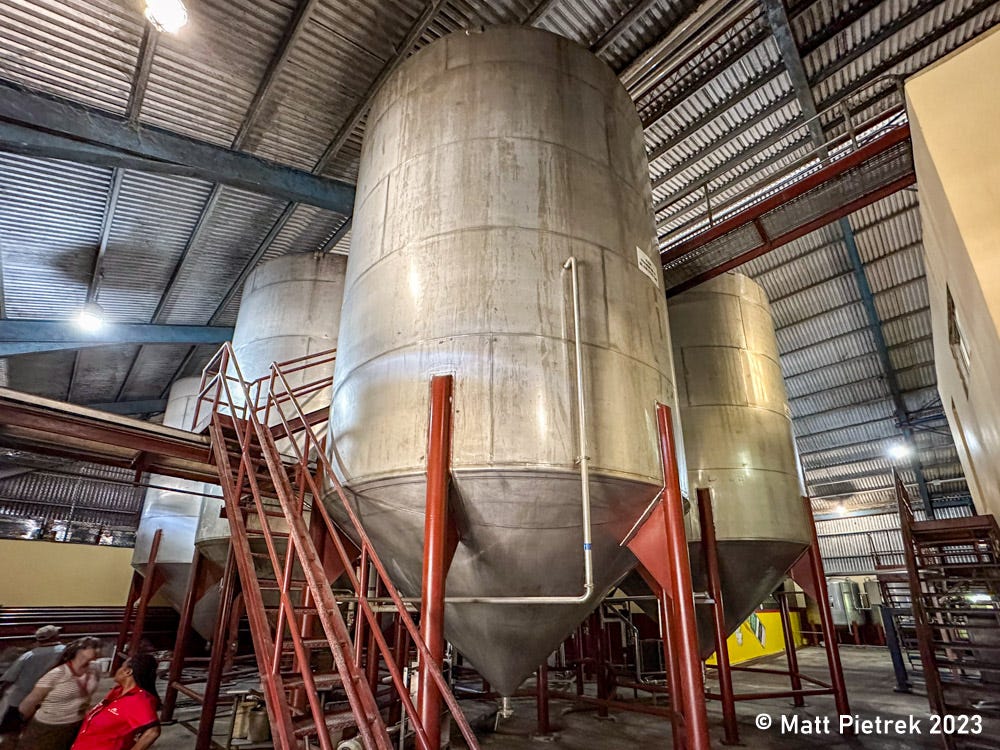This detailed color photograph, taken by Matt Pietrek in 2023, captures the interior of a vast, industrial warehouse or manufacturing facility. The structure features corrugated metal walls and ceiling, supported by striking blue steel I-beams. Dominating the scene are six enormous, stainless steel vats or tanks, reminiscent of those used in breweries. These tanks, conical at the end, are elevated on red metal legs with matching stair railings leading up to their tops. A series of metal stairs and walkways crisscross between the tanks, adding to the intricate industrial aesthetic. 

In the lower right corner, the floor space is populated by three people wearing lanyards, likely surveying or performing tasks in the facility. The concrete floor extends to integral office-like buildings within the larger structure. Additional smaller tanks and large hoses can be seen scattered in the background. The image's orientation is slightly wider than tall, encapsulating the sheer scale and complexity of this industrial or agricultural production environment.